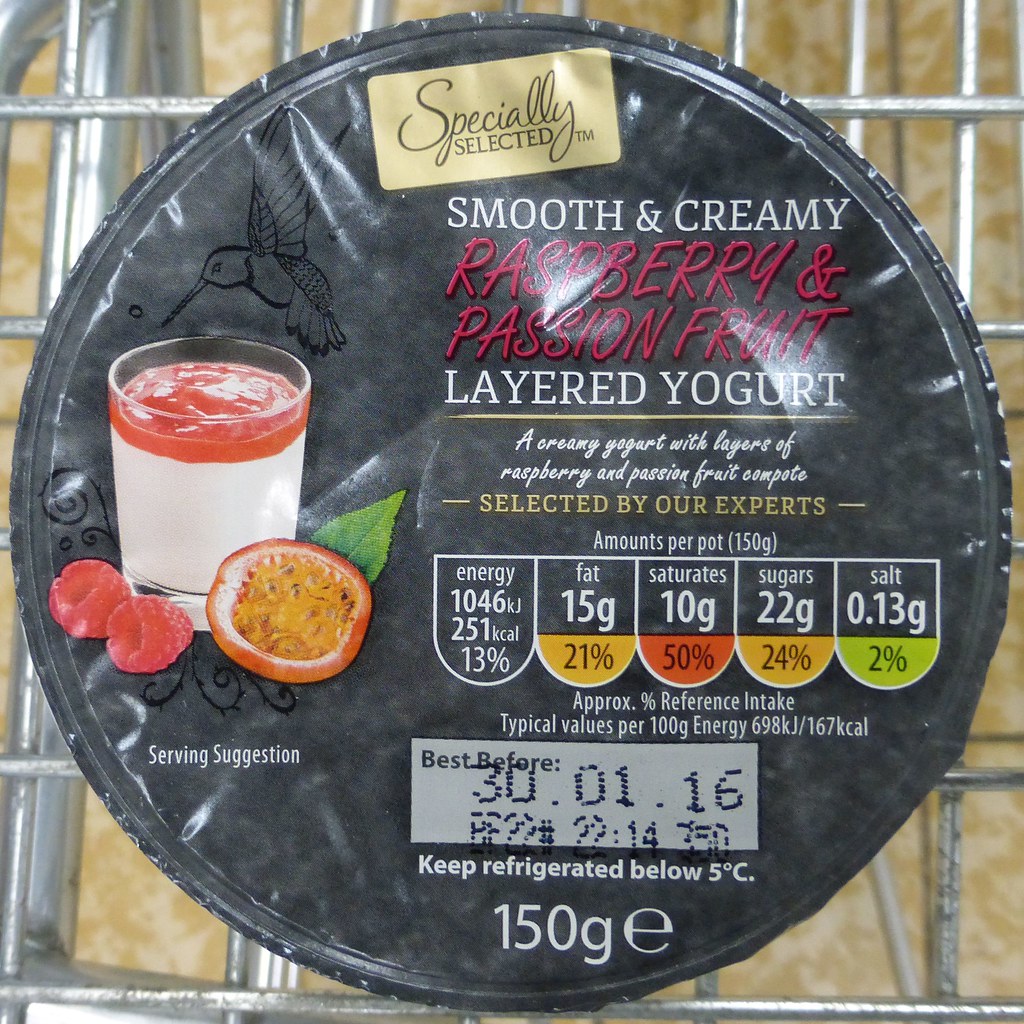This close-up photograph features a container of "Specially Selected" smooth and creamy layered yogurt with a black circular lid adorned with intricate images and designs. At the very top of the lid, a gold rectangular strip displays the "Specially Selected" trademark. Beneath, in white text, it reads "Smooth and Creamy". Then in vibrant red text, it highlights the flavor "Raspberry and Passion Fruit", followed by "Layered Yogurt" in white. Just below, a yellow line divides the descriptive text: "A creamy yogurt with layers of raspberry and passion fruit compote", along with the note "Selected by our experts" in yellow text flanked by dashes. 

Further details include nutritional information such as amounts per pot (150g), energy (146 KJs/251 calories - 13% of daily intake), fat (15 grams), saturates (10 grams), sugars (22 grams), and salt (0.13 grams). The product is best before January 30th, 2016, and should be kept refrigerated below 5°C. 

Alongside the text on the left side of the lid is an image of a glass jar filled with creamy white yogurt topped with yellowish and reddish raspberry and passion fruit compote. 

The container is situated in a metal shopping cart, indicating that it was taken in a shopping environment, likely a grocery store or a café.